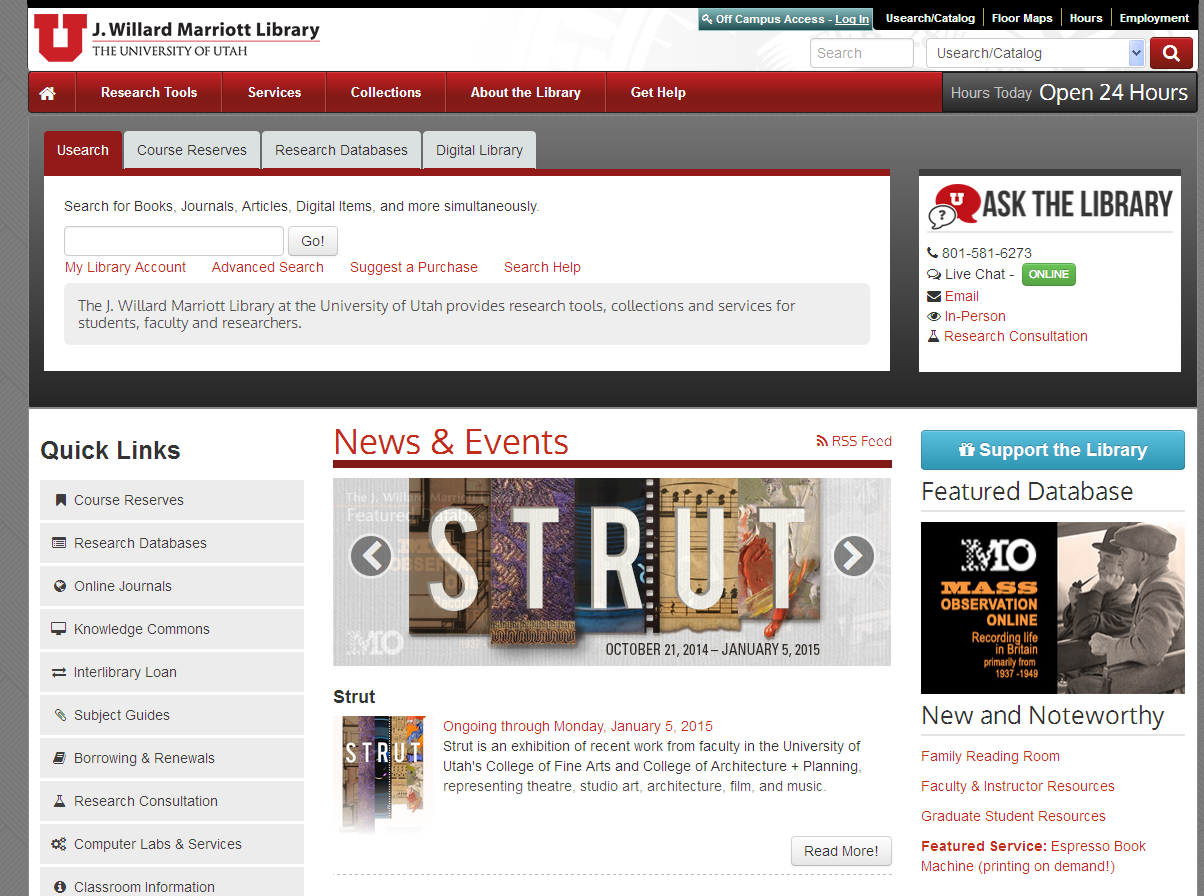The image depicts the homepage of the J. Willard Marriott Library on the Stanford Utah University website. The background features a combination of dark gray, black, and white colors. At the top left corner, the name "Stanford Utah University" and "J. Willard Marriott Library" are prominently displayed. Adjacent to this, there's a menu that includes options for off-campus access log-in, research catalog, formats, hours, and employment.

Below this, there are two important boxes: one for the search bar and another for the research catalog with a drop-down menu. Further down, a maroon-colored menu bar offers links to research tools, services, collections, information about the library, and help services. The statement "Open 24 hours" is also clearly noted.

Another tabbed menu sits beneath this, providing even more options. A prominent search bar follows, where users can look for books, journals, articles, and other resources. Right next to this search bar is a contact box titled "Ask the Library," which includes a phone number, live chat option, email, and information for scheduling research consultations.

The bottom half of the page is divided into several sections. To the left, there is a "Quick Links" menu with options for accessing journals, research databases, and subject guides. Next to this is a section for news and events, featuring an image and description of an exhibition titled "STRUT," which was scheduled to run from October 31, 2014, to January 5, 2015.

In the bottom right corner, a "Support the Library" section invites users to explore various ways to support the library, including possible donations and online observations.